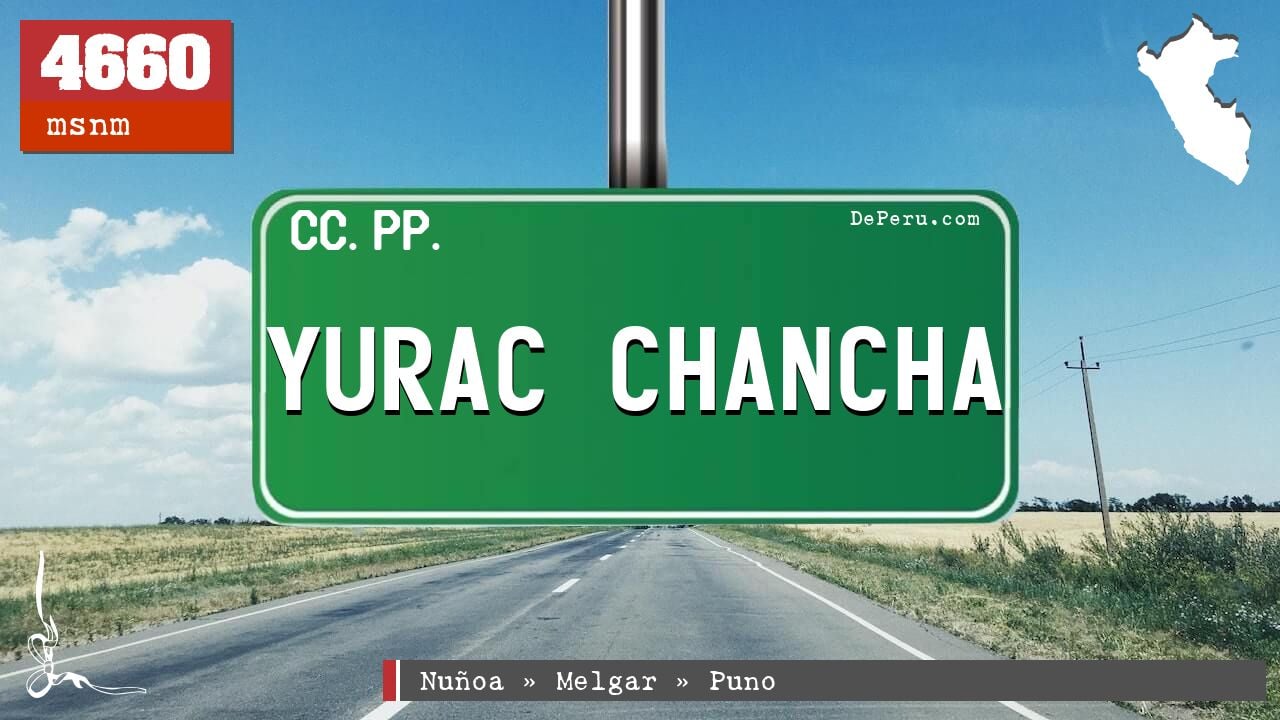The image depicts a detailed and vibrant scene of a country road flanked by grassy fields, extending diagonally from the bottom corners towards the horizon. Centrally prominent in the image is a green license plate suspended from a thick metal bar, adorned with a white border and inscribed with cc.pp in the top left corner and deperu.com in the top right. Boldly across the plate are the letters “YURAC CHANCHA” in large white font. The top left features a red rectangle with the inscription "4660 MSNM" in white, while the top right corner displays a white silhouette of what appears to be the country of Peru. At the bottom of the image is a gray bar, with white text listing "NUNOA," "MELGAR," and "PUNO," interspaced with small arrows. There's also an indistinct white symbol at the bottom left, further emphasizing the detailed and layered nature of the scene.